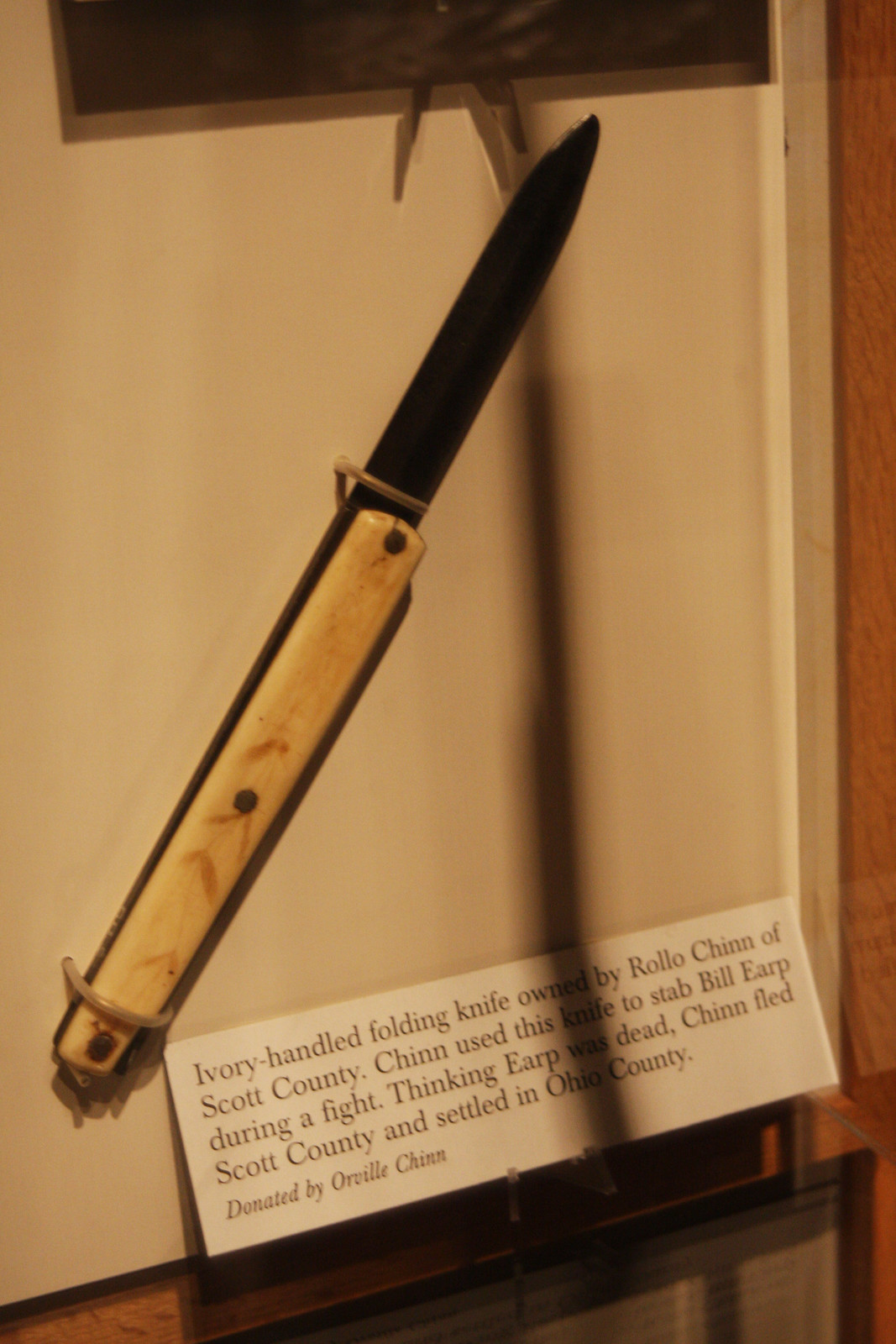The image showcases an ivory-handled folding knife prominently centered and tilted at a 45-degree angle against a white wall. Secured by transparent plastic supports, the knife appears to be part of a historical exhibit, possibly in a museum. Below the knife, a white placard with black text provides detailed information about its provenance and historical significance. The text reads: "Ivory Handled Folding Knife owned by Rolo Chin of Scott County. Chin used this knife to stab Bill Earp during a fight. Thinking Earp was dead, Chin fled Scott County and settled in Ohio County. Donated by Orville Chin." The background features a light brown wooden base and a white wall, emphasizing the knife's historical artifact status.